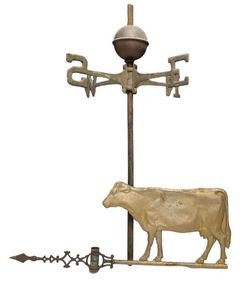The image showcases an elaborate weather vane, prominently featuring a large, golden cow positioned near its base. The cow, facing to the left, stands atop a horizontal rod. The weather vane itself is crafted from a dark metal, possibly brass. Above the cow, there is a vertical rod that culminates in a spherical object at the very top. The rod also supports directional indicators for north, south, east, and west, with south and east being especially prominent in this photograph. A spear-like point extends from the top of the weather vane, designed to show the direction of the wind. The detailed and ornate design suggests it might be an ornamental piece, possibly made for a ranch. The entire structure is set against a plain white background, highlighting its intricate features.